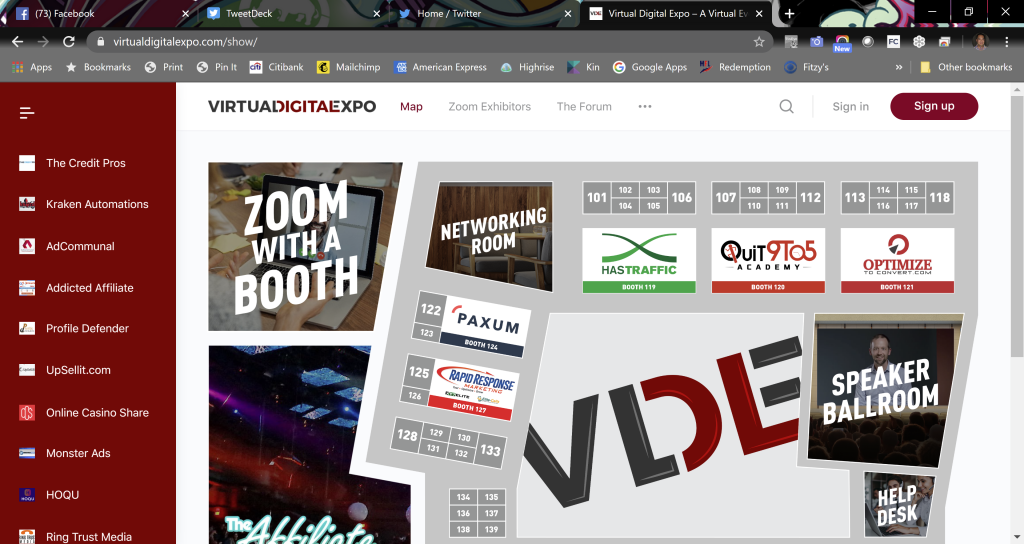This image depicts the screen of a laptop displaying a browser with multiple tabs open. At the top of the browser, several tabs are visible, which include Facebook, two separate tabs for Twitter (one being the Twitter homepage), and a virtual digital expo tab. The currently active tab is the virtual digital expo.

The left sidebar of the screen is highlighted in red, listing various participants and companies such as The Credit Pros, Kraken Automations, AD Communal, Addicted Affiliates, Profile Defender, upsalt.com, Online Casino Share, Monster Ads, HOQ, and Ring Test Media.

Dominating the center of the screen is the Virtual Digital Expo logo. Below the logo, there are multiple images arranged in an irregular layout. Some of the visible sections include "Zoom with the Booth," "Networking Room," "Speaker Ballroom," "Helpdesk," "The Affiliates," "Paxam," "Quiet9205" or "Quiet9205," "Optimize," and "House Traffic." The screen as a whole appears to be part of a virtual event or exhibition platform.